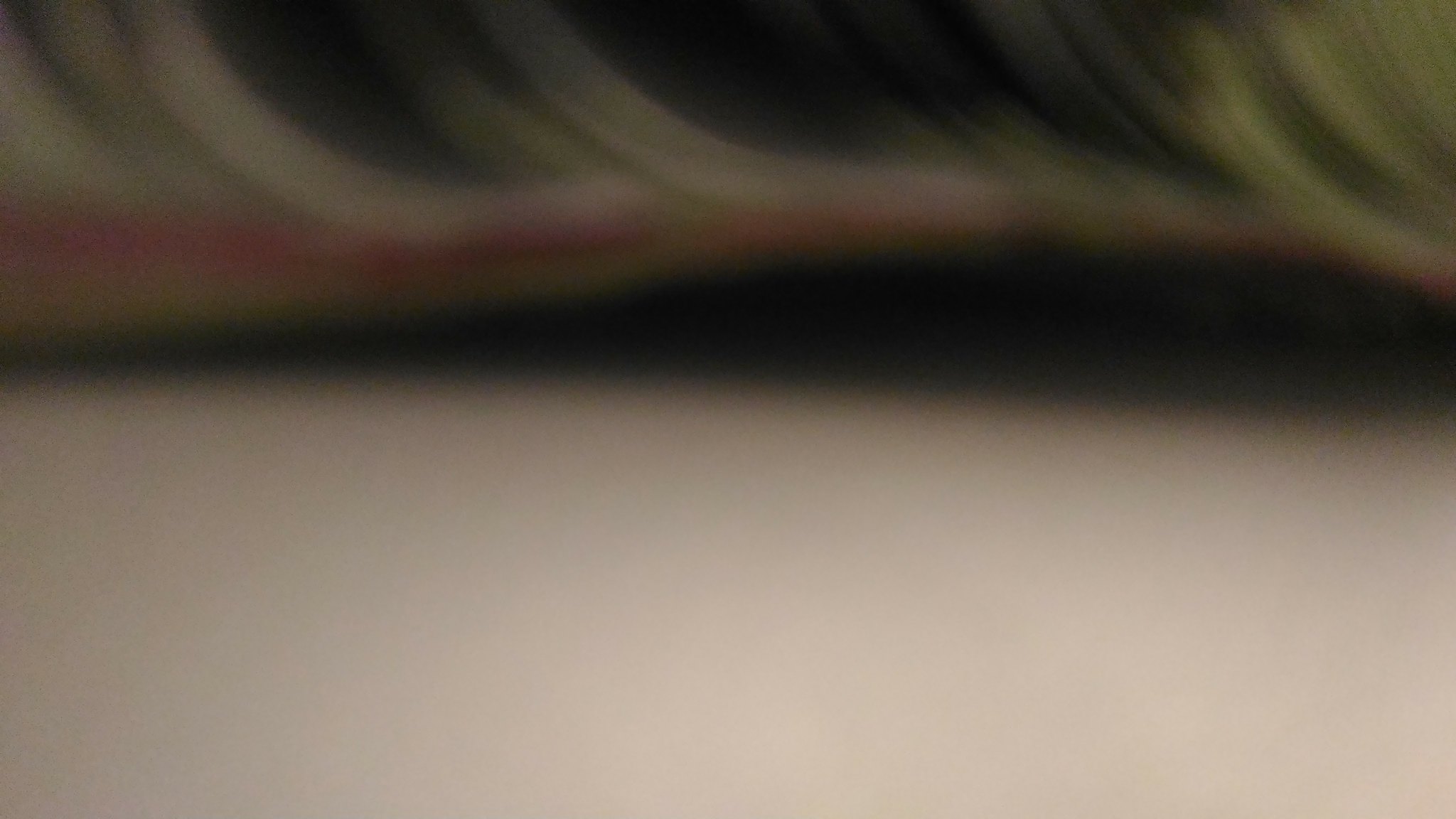The image depicts a scene with a white ground that could be snow or a blank surface. The top part of the image features what appears to be a dark, roof-like structure or possibly a magazine cover, with slipped black elements. There are white lines running across this section. In the middle of the image, there is a brown area with darker brown edges and some black, though the scene is very out of focus, making it hard to distinguish details. The overall impression is vague due to the blurriness, leaving the specific subject matter difficult to identify.